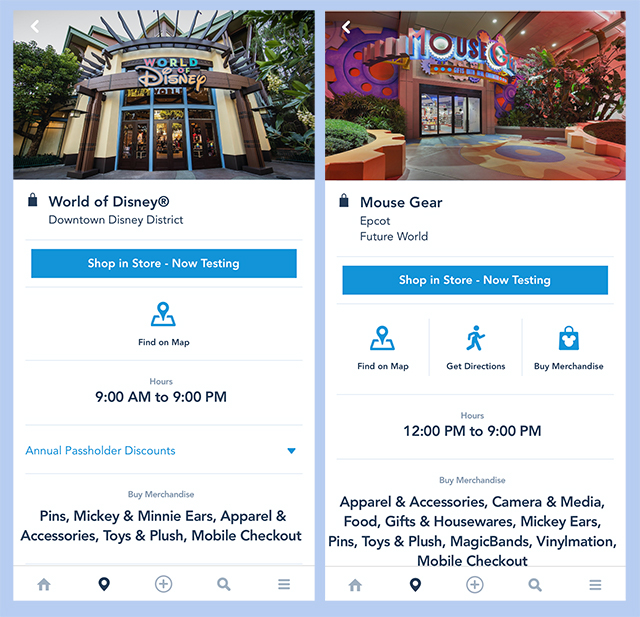The image depicts two distinct mobile screenshots, both characterized by a light blue background. On the left screenshot, the upper left corner showcases an image labeled "World of Disney," indicating either a Disney attraction or store. The vibrant text varies in color and size: the 'W' is capitalized in red, the 'O' in blue, the 'R' in lime green, the 'L' in yellow, and the 'D' in blue. The word "of" follows, with the 'O' in smaller red and the 'F' in smaller yellow. The iconic Disney logo appears in orange. Below this, on the left side, there is a dark gray or black padlock icon. Adjacent to it, "World of Disney®" is written in bold, with a registered trademark near the 'Y.' Beneath this, in smaller black text, it reads "Downtown Disney District." Two faint blue lines act as dividers, with a section in the center featuring a rectangular blue background. In bold white text, it reads "Shop in Store – Now Testing."

The screenshot on the right features an image at the top of a building with whimsical design elements and the partially visible word "Mouse," which seems to end with a 'G' that gets cut off. The 'M' is tall and pink with an ombre gradient transitioning from light to dark pink, while the 'O' resembles a ring adorned with studded diamonds. The building's front facade features at least two, but possibly four, doors and floors with gear symbols. Below this image, on the left side, there is a gray padlock icon. To the right, in bold, it says "Mouse Gear."